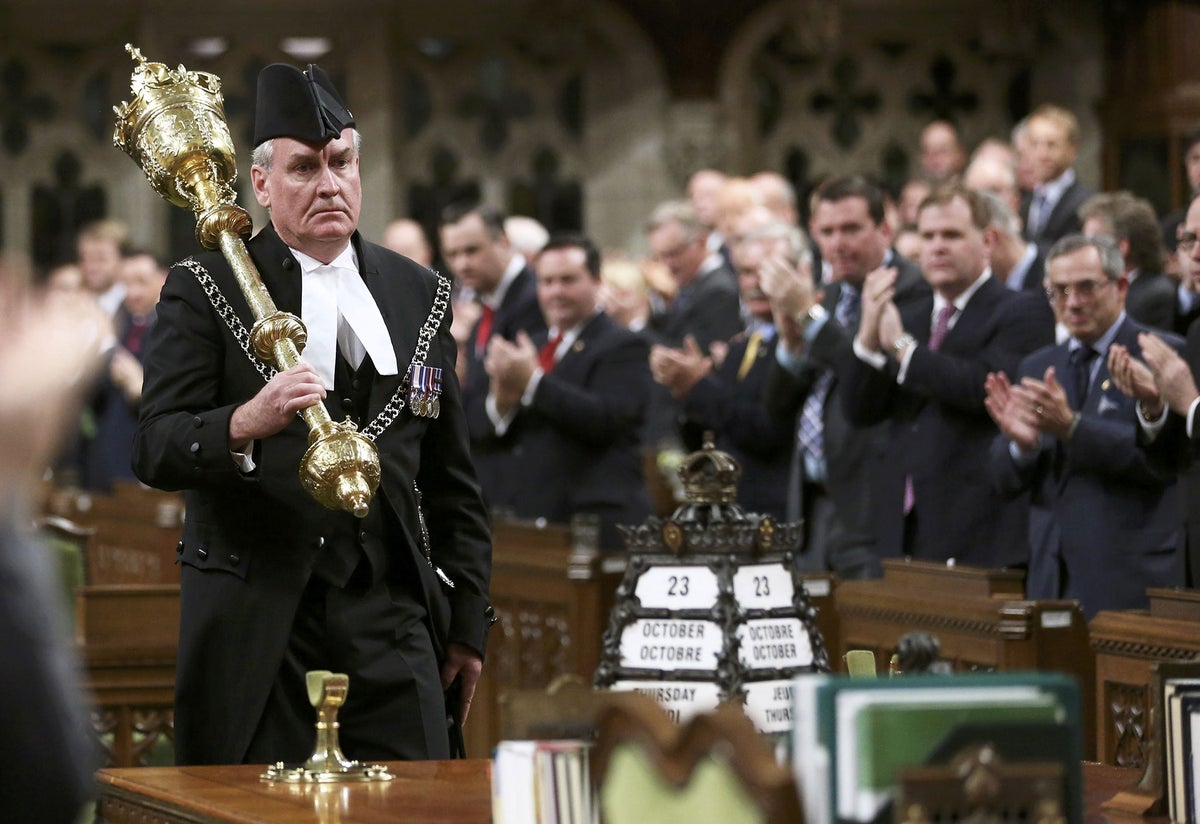In the interior of what appears to be the British Parliament building, a solemn-faced gentleman stands prominently, dressed in a formal black uniform complete with a long black jacket, black pants, and a black hat with a pointed front and narrow back. A white collar with an ornate ribbon hanging down contrasts sharply against his dark attire. Several military ranking ribbons adorn his chest. He holds a large golden rod, crowned at the end, resting on his shoulder. In front of him, a table displays a sign marked "23rd of October" and a brass candle holder, possibly awaiting the candle he carries. The background reveals an assembly of men in professional dark suits, all standing behind wooden barriers, clapping in acknowledgment of the man’s presence and actions.